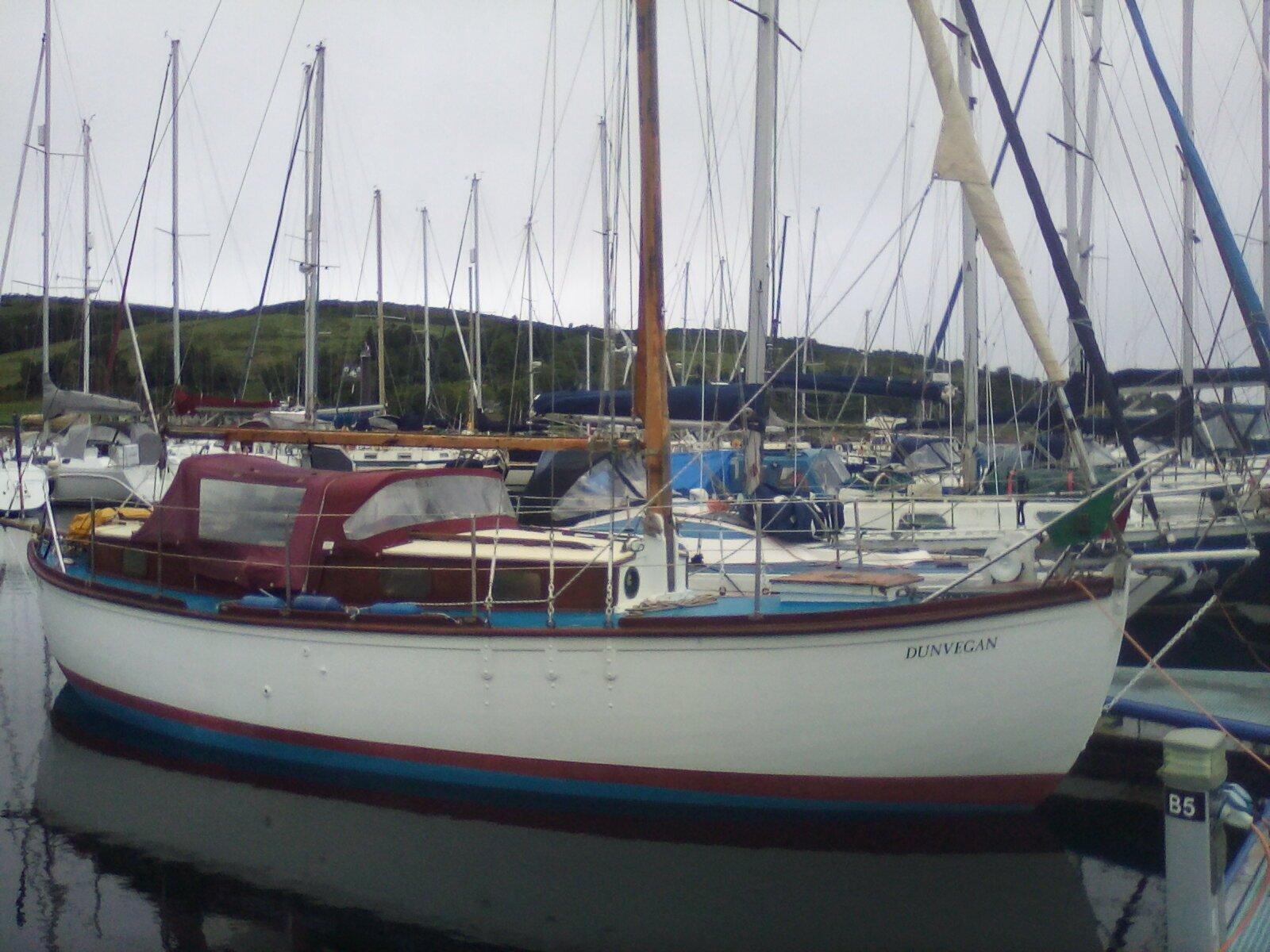This outdoor daytime photo captures a bustling harbor with numerous docked sailboats, their masts prominently piercing the gray sky. In the foreground, the sailboat 'Dunvegan' stands out, boasting a white hull detailed with burgundy stripes near the top and bottom, where it meets the water. The boat's enclosed cabin is also adorned in burgundy. The name "Dunvegan" is painted on the hull in stark white letters. To the right, a post marked B-5 suggests a docking position. The background features rolling hills, adding a serene contrast to the busy dock, where a multitude of boats are anchored, all with sails down and rigging in view.